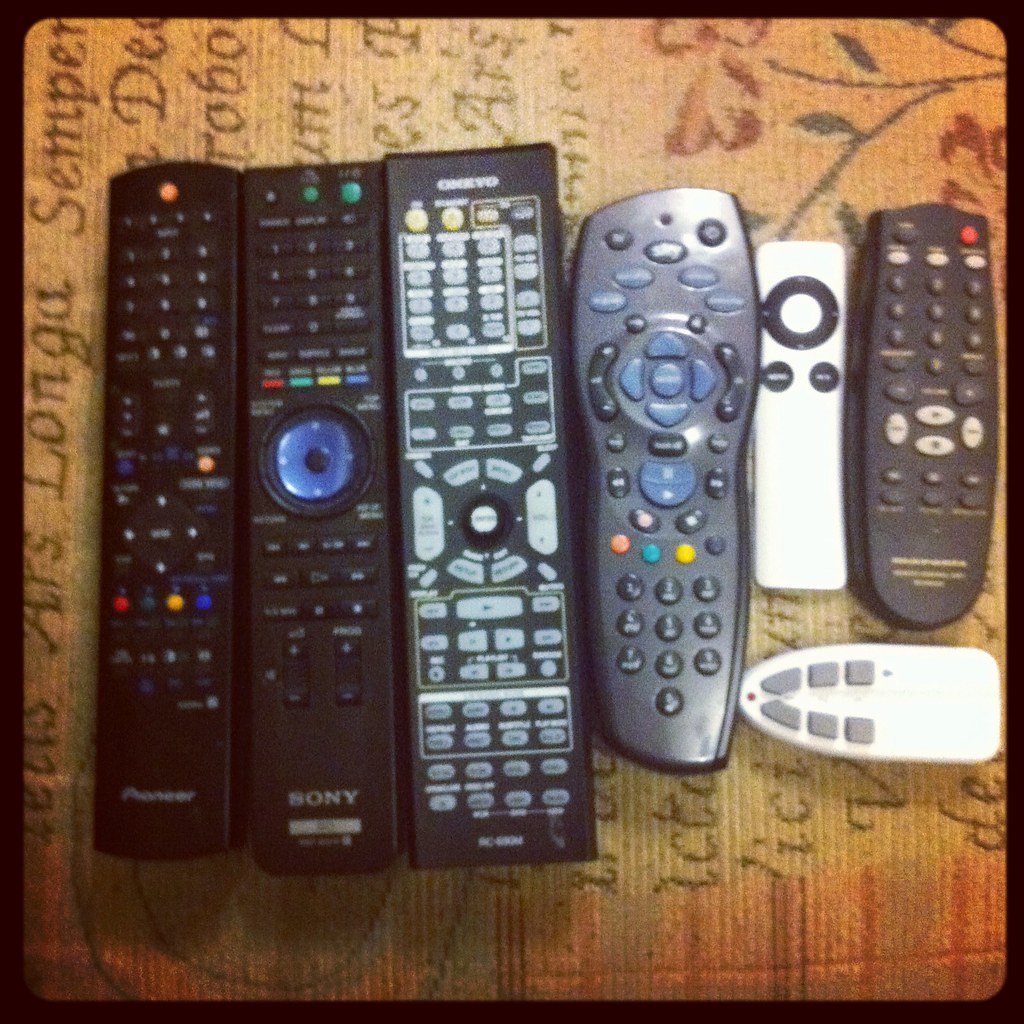The photo features seven remote controls arranged on a rug with intricate designs and etched writing. The majority of the remotes are black, with a couple in silver and one significantly smaller, white remote belonging to an Apple TV. Large multi-device television remotes branded as Pioneer, Sony, and Onkyo are on the left, characterized by numerous buttons including numpads. Adjacent to these is a TiVo remote, distinguishable by its directional buttons at the top. 

Next, the Apple TV remote stands out with its minimalist design, featuring an iPod-like navigation pad instead of a numpad. To the right of the Apple TV remote, a smaller, black television remote and an unbranded, short white remote with six buttons are positioned, the latter lying horizontally.

The background rug or mat underneath these remotes has decorative motifs, with visible art including red petals and green leaves among the writing, giving a textured and artistic backdrop to the varied shapes and functionalities of the remotes.